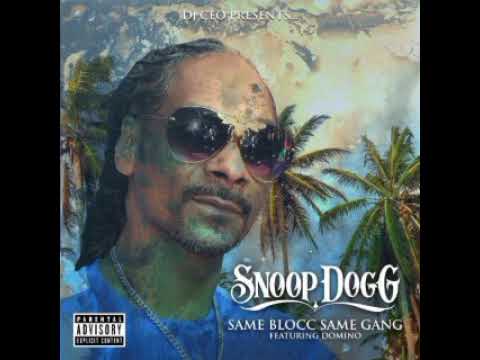This image is an album cover featuring the iconic rapper Snoop Dogg. Framed by thin black bars on both the left and right sides, the central square showcases an illustrated backdrop with a blue sky, palm trees, and clouds. At the forefront, Snoop Dogg stands out, looking directly at the camera. He's depicted as a slender, light-brown-skinned man with a distinctive black goatee and shoulder-length hair that's grayish on top and black at the ends, hinting at a balding hairdo. He is wearing large, tinted black aviator sunglasses, a blue t-shirt, and a thin silver chain necklace.

Above his head on the left side, the text reads "Dr. CEO presents." Towards the right, in white letters, it says "Snoop Dogg, Same Block Same Gang, featuring Domino." A Parental Advisory Explicit Content sticker is prominently placed in the lower left corner. The album cover's design, colors, and elements strongly suggest it as a front cover for a musical CD, with shades of blue, black, white, gray, brown, and green setting the tone.